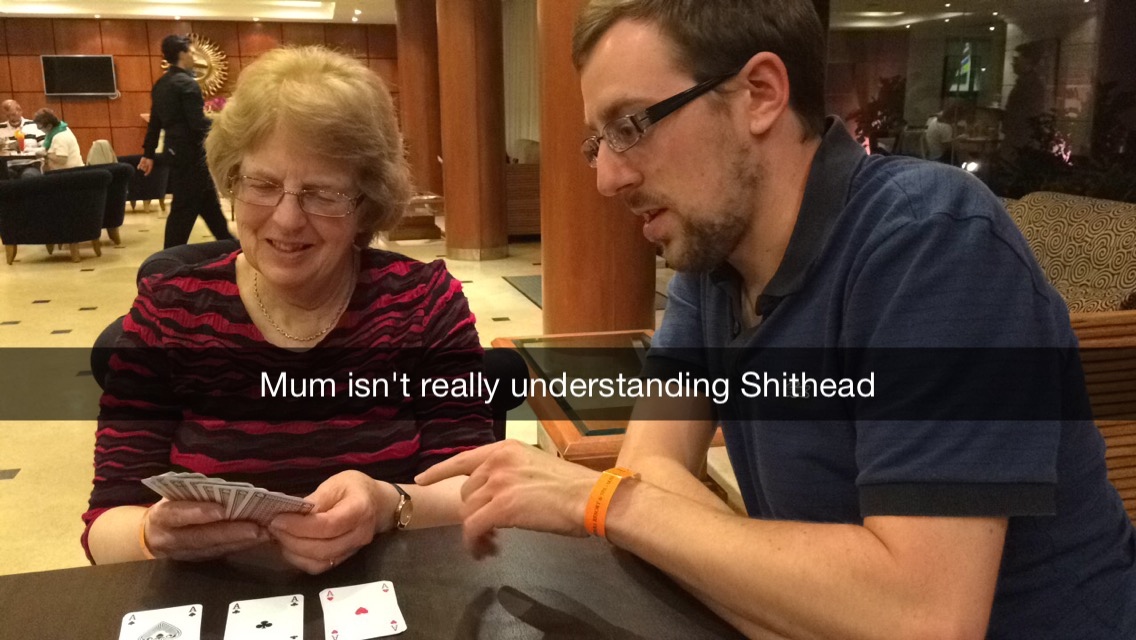In a cozy setting that appears to be a bar, café, or hotel lobby, an older lady and a younger man are engaged in a game of cards. The image features a caption across the center, horizontally set against a black background line with white text that reads, "Mum isn't really understanding Shithead." Shithead, likely the name of the card game, is highlighted with a capital letter.

On the left side of the photo, the older lady has short, blonde to light brown hair and is wearing glasses. She has a warm, smiling expression and dons a red and black wavy striped top. A watch adorns her left wrist, and she is holding cards that face away from the camera. On the table in front of her are three piles of cards, clearly visible are the ace of spades, ace of clubs, and ace of hearts.

To the right, the younger man with short brown hair also wears glasses, which have thick black arms. He is dressed in a short-sleeved navy polo shirt and wears an orange event bracelet on his left wrist. In the background, the ambiance is lively with other patrons seated at tables and what seems to be a waiter walking past on the tiled floor.